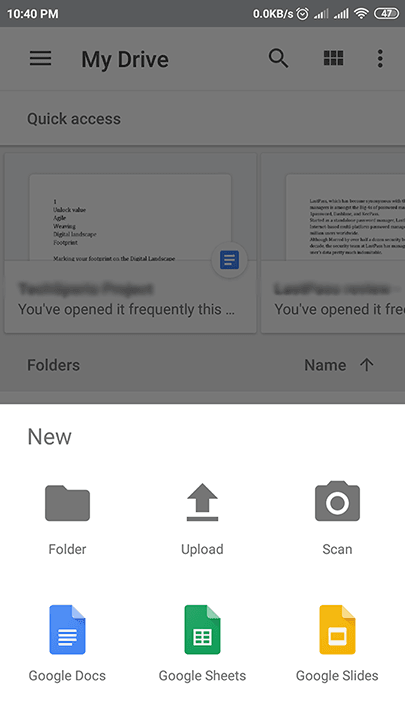A cell phone display showing the Google Drive interface at 10:40 p.m. is depicted. At the top of the screen, within a gray notification bar, various indicators are present: the time "10:40 p.m." on the left, followed by "0.0 kV/s", an alarm icon, cell signal bars, a Wi-Fi icon, and a battery indicator at "47%". 

Below the notification bar, the screen is overlaid with a semi-transparent gray background. The main interface showcases several icons and options: three horizontal lines stacked indicating a menu, followed by icons representing "My Drive," a magnifying glass for search, a grid of six boxes for apps, and three vertical dots symbolizing more options. The section titled "Quick Access" is noted, though parts of the content are blurred, with a hint suggesting frequent use of certain folders.

Located underneath is a distinct section featuring a white background with black text. This section displays icons for creating new content: a folder icon, an upload icon, a scan icon resembling a camera, and icons for Google Docs, Google Sheets, and Google Slides, each in their respective colors—blue, green, and yellow. The general color scheme throughout the screen includes shades of gray, but excludes true black, emphasizing slate gray tones instead. The overall impression is that the user is navigating through their Google Drive, accessing folders and various file creation options within the interface.